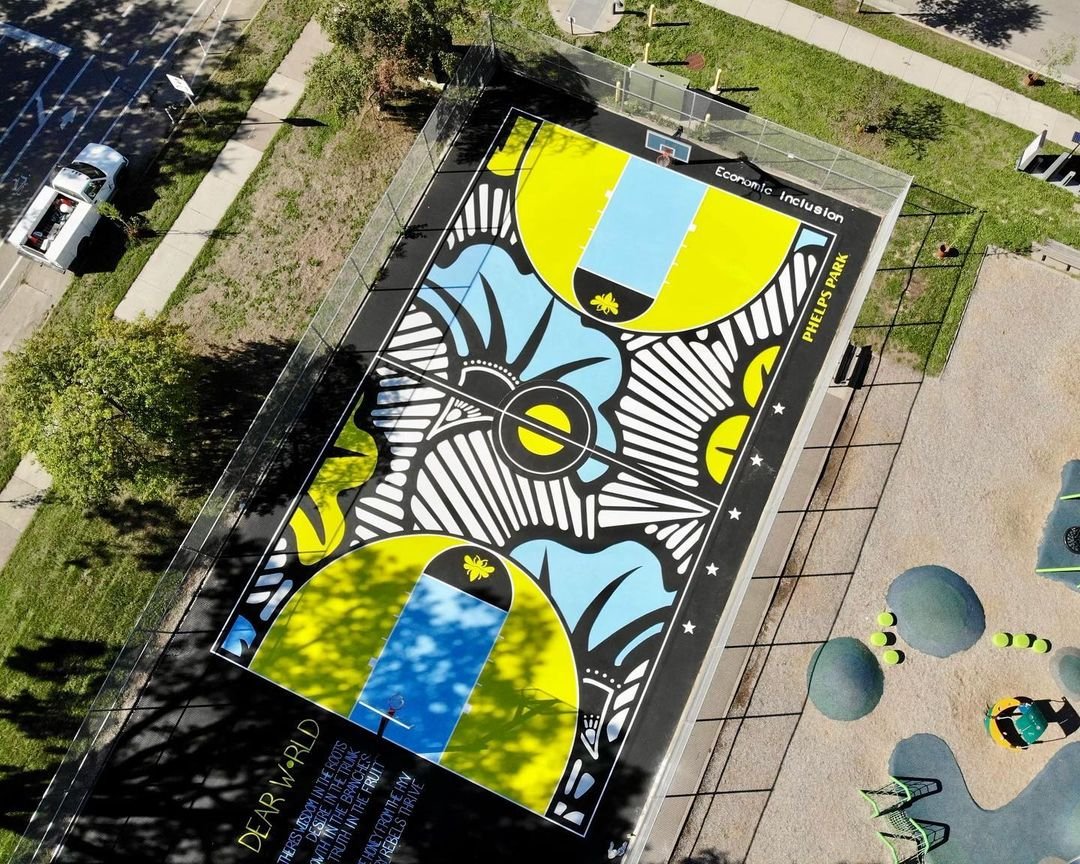This aerial photograph captures an urban scene centered around a vibrantly painted basketball court, surrounded by strips of grass, sidewalks, and a street with a white truck. The court itself is a striking mosaic of colors: black, white, light blue, dark blue, and a vivid yellow. Dominating the court's artwork are bold, black outlines reminiscent of a coloring book. Key features include a light blue key area, a black semi-circle above the free-throw line adorned with a yellow bee, and a black and white central design flanked by yellow arcs within the three-point lines.

Inscribed along the shorter sides of the court is "Economic Inclusion," while the longer sides are marked with "Phelps Park" in yellow. An adjacent area outside the court displays chalkboards with the message, "Dear World, there's wisdom in the roots, desire in the trunk, growth in the branches, and truth in the fruit. Honey from the hive, rebels thrive," and additional partially visible text.

To the side of the court, a small playground features climbers and other interactive structures, complementing the community-focused setting of this unique and colorful urban sports venue.